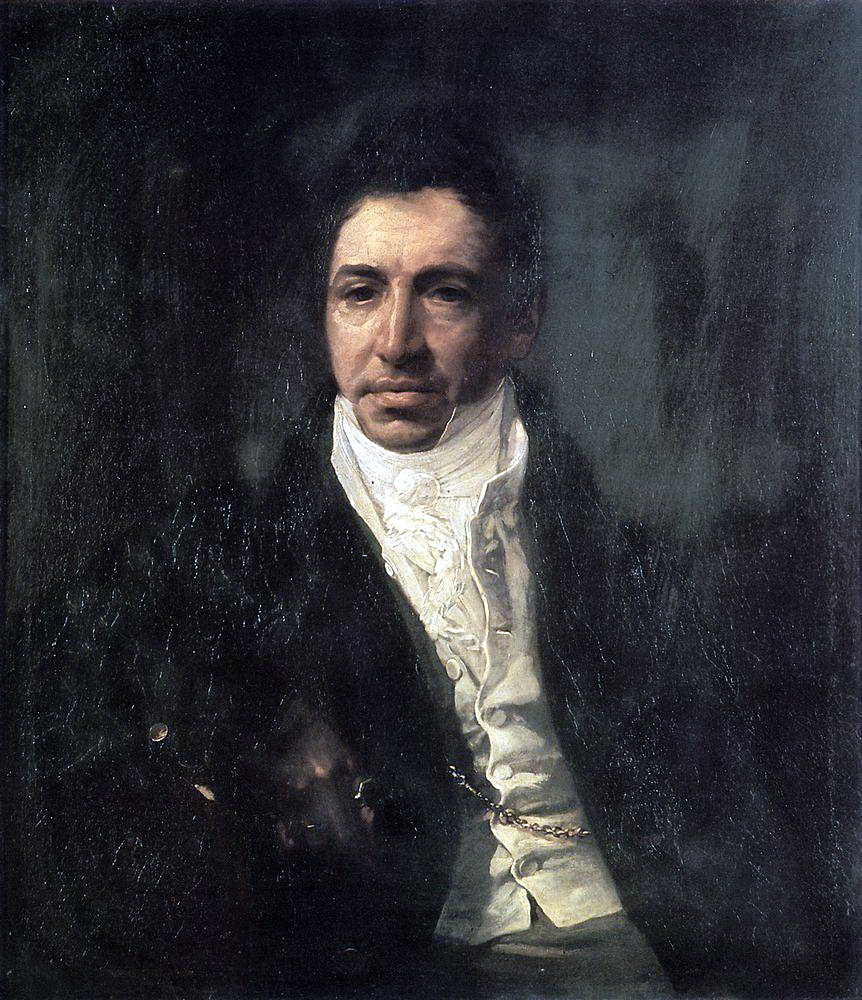This detailed portrait appears to be an artistic rendering, possibly of a historical figure such as Russian General and Secretary of State Pyotr Kikin, painted in an old style with evident age-related wear like cracking and flaking paint. The man in the portrait is depicted with short, dark hair and dark eyes, and he has a neutral expression on his face. He wears a black coat that blends into the dark background, making it challenging to distinguish where the coat ends and the background begins. The coat is adorned with fancy gold buttons and features a chain, possibly an old-fashioned watch chain, across the waist. Beneath the coat, he wears a elaborately patterned white shirt with ruffles and buttons up the front, and a white neckerchief tied around his neck. The man is slightly facing to the right side of the image, with his head turned in that direction, and his mouth firmly shut. Notably, his left ear is visible while his right ear is not. The backdrop consists of flowing tones of gray and white, enhancing the somber and historic ambiance of the portrait. There is a hint of what might be his right hand, possibly gloved, resting on an unseen object. Overall, the main colors in the composition are gray, black, and white, contributing to its stark yet dignified appearance.